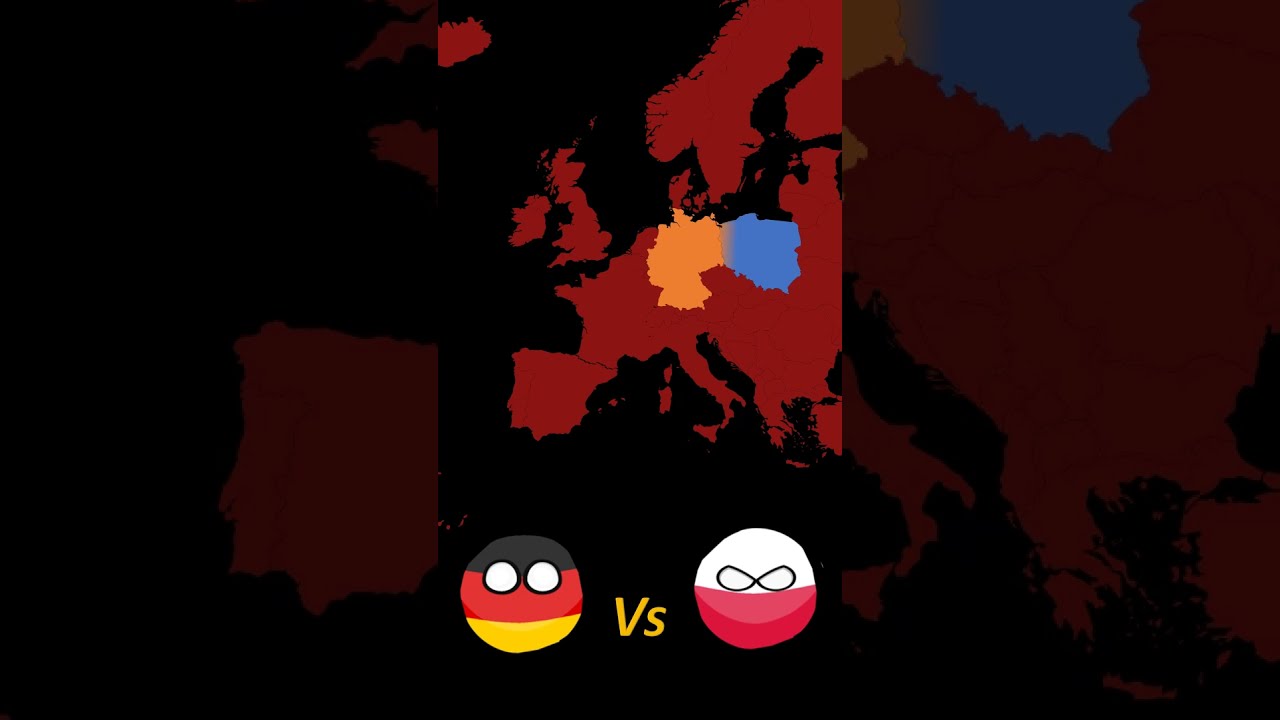The image is a computer graphic divided into three segments. The outer segments on the left and right are darkened, resembling an overlaid filter, while the central segment features a detailed, stylized map of Western Europe rendered in red and black colors. Germany is highlighted in orange and Poland in blue within this red landmass. The background behind the map mimics darker, zoomed-in portions of the same map. Below the map, two emojis face off, representing Germany and Poland: the German emoji features the national flag colors—black, red, and yellow—with wide eyes, whereas the Polish emoji displays white and red horizontal stripes and has goggle-like eyes. Between the two emojis is the word "Versus" in yellow text. The entire image invokes a sense of a video game interface where two countries are competing.